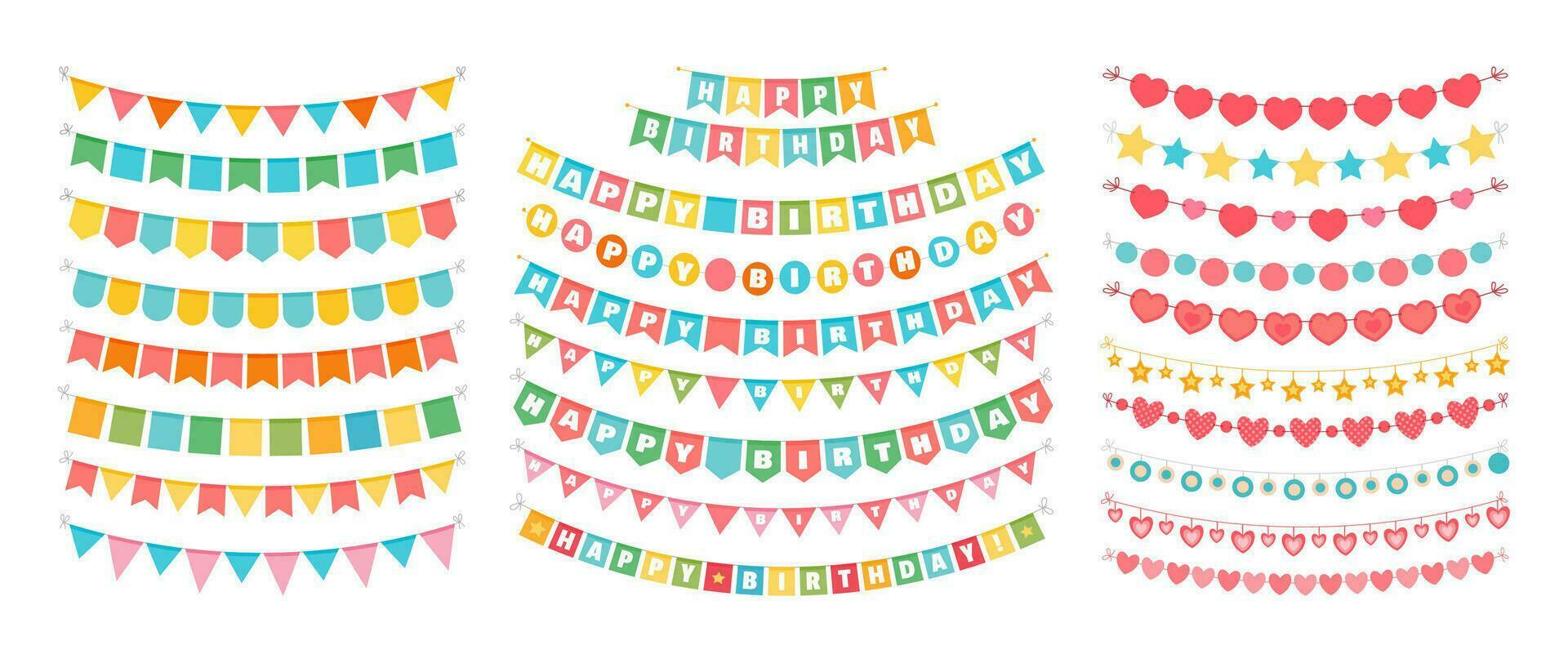This image is a horizontally rectangular, multi-colored print piece with no border, set against a white background. It comprises three vertically rectangular sections, each showcasing different styles of celebratory flags, presumably for a birthday event. 

On the left section, various flag designs are displayed, including triangular, square, upside-down house-shaped, and upside-down arch-shaped flags. These flags come in multiple colors, providing a diverse visual assortment.

The middle section features a banner that spells out "Happy Birthday" across different flag designs. Each letter is presented on a unique flag with varying shapes and colors such as blue, yellow, red, green, and orange, making the banner festive and vibrant.

The right section displays a pattern of banners with repeating motifs of hearts, stars, and circles. The colors for these flags predominantly include red, yellow, and blue. The sequence of shapes starts with hearts, followed by stars, circles, and then repeats several times.

Overall, the image appears to be an advertisement showcasing a pack of birthday banners available for purchase, illustrating the diverse styles and designs included.